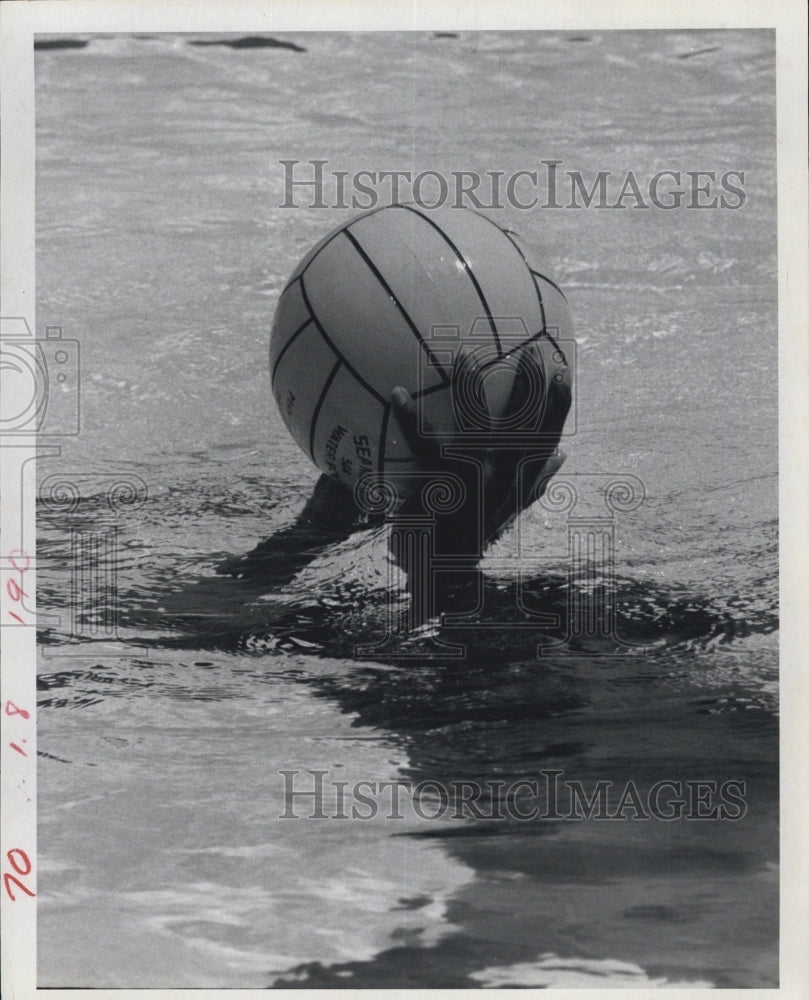In this black-and-white photograph, we are given a strikingly close-up view of a serene, water-based scene where two hands of a person with relatively dark skin protrude from the water, centrally positioned while holding a volleyball aloft. The image captures only the water and hands emerging with the volleyball, causing the significant detail of the player’s position inferred to be facing roughly the 8 to 9 o'clock direction. A shadowy figure is vaguely visible beneath the water's surface.

Translucent text on the image reads "Historic Images," appearing twice—once above and once below the volleyball. Additionally, there is a faint design featuring ancient Roman columns and a traditional film camera nestled on a pedestal partially overlaying the hands and volleyball. The left side of the image includes faintly visible numbers: 70, 1.8, and 190. This image, reminiscent of an old photograph or magazine page, contains watermarks subtly visible on the paper, contributing to its vintage feel.